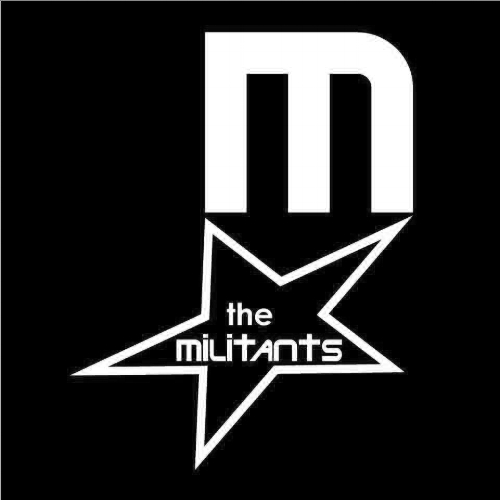The image features a logo set against a solid black square background. Prominently positioned in the upper right corner is a bold, white letter "M." Directly beneath this, there is a five-pointed white star. The star is asymmetrical, with one of the points extending farther to the right, creating a somewhat human-like shape with the side points resembling arms and the lower points like feet. Inside the star, in a simple, non-formal font, are the words "The Militants," with the letter 'T' notably styled to resemble a cross, and the word "THE" in lowercase. The overall design suggests it could be an advertisement or album cover for a band called "The Militants," characterized by its straightforward black and white color scheme and minimalist design, potentially indicating an amateur creation.